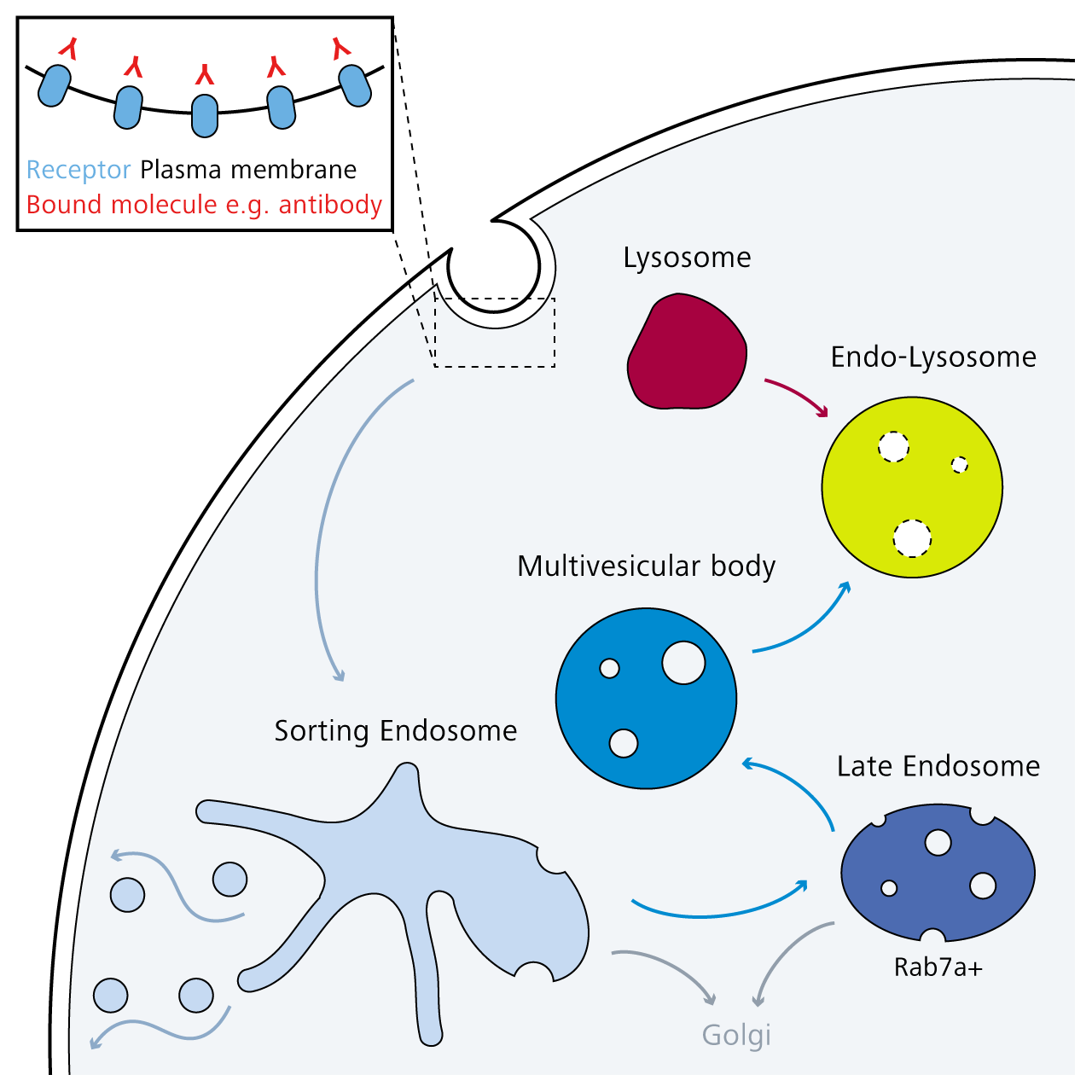The image is a detailed multicolored educational print piece, primarily focused on a cellular diagram. In the upper left-hand corner, there's a rectangular box with a black border, displaying a close-up of five bluish pill-shaped structures, each adorned with red ribbon-like elements, labeled "Receptor Plasma Membrane Bound Molecule e.g., Antibody." The main part of the diagram appears to depict a partial cell, shown as an arc from the bottom left to the top right, which contains several distinct organelles and structures. In this arc-shaped section, various components are identified: a red, circular shape labeled "Lysosome" sits towards the top; a lime-green, round shape labeled "Endolysosome" is positioned to the lower right; and a blue circular structure labeled "Multivesicular Body" is located more centrally. Additionally, there are other labeled elements such as "Sorting Endosome," "Late Endosome," and various arrows indicating interactions and pathways among these structures. The image appears to be designed for scientific educational purposes, likely aimed at explaining cellular organization and function.